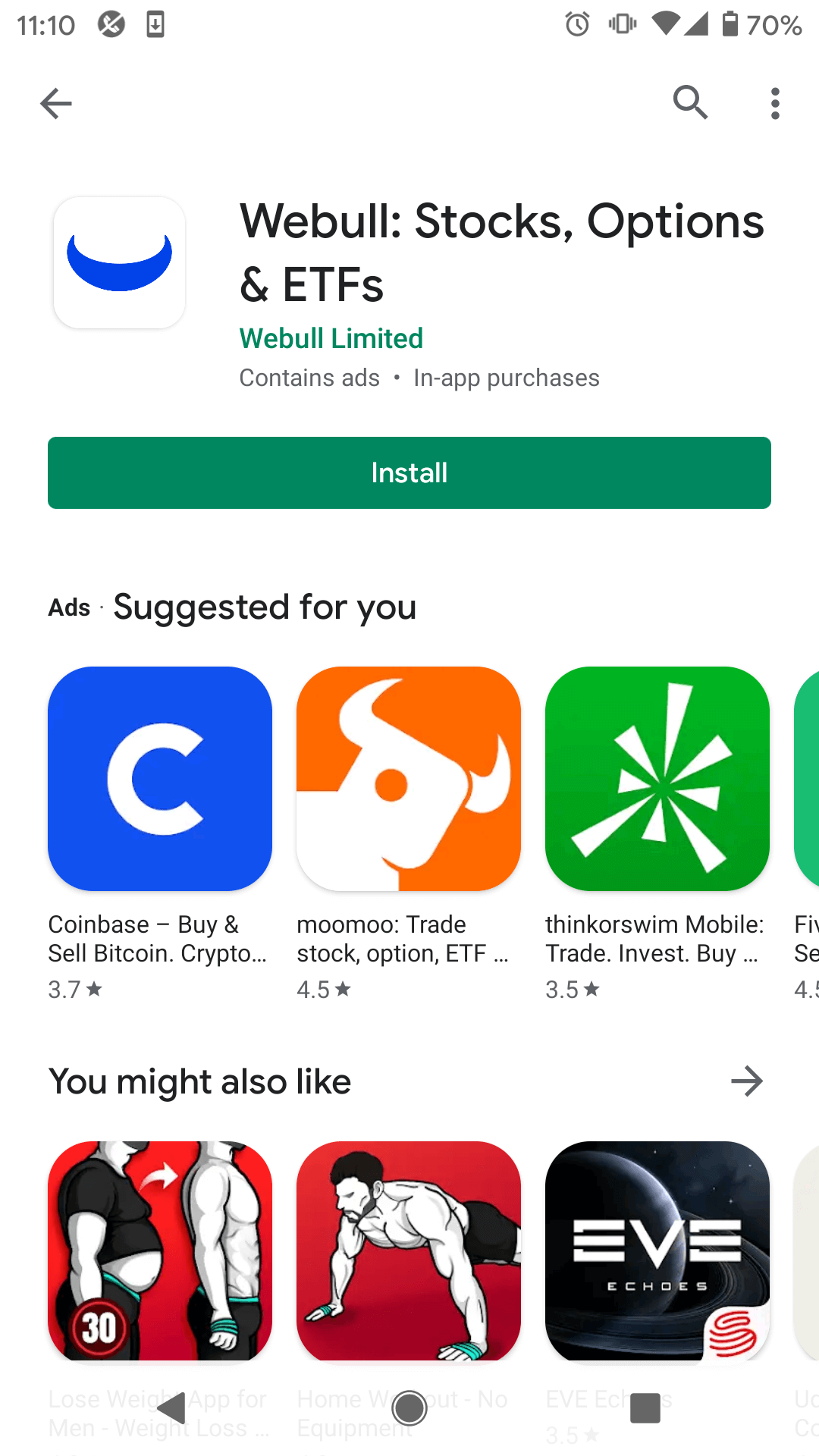**Detailed Caption for the Screenshot:**

The screenshot shows the Google Play Store interface on an Android device. 

**Top of the Screen:**
- The status bar at the top is in grey, displaying the time as 1:10.
- Various icons are present, including a "Do Not Disturb" icon, a system download icon, an alarm icon, a vibrate icon, Wi-Fi and cellular network indicators, as well as a battery icon with the battery percentage at 70%.

**Main App Information Section:**
- Below the status bar, the background is white.
- On the top left is a back arrow. To its right are a search button and a three-dot menu button.
- After some blank space, a logo appears on the left. The logo features a blue eclipse shape with a grey outline on a white background.
- Next to the logo, bold black text reads "Webull: Stocks, Options, and ETFs."
- Underneath the title, in green text, it says "Webull Limited."
- Further below in smaller grey text, it states "Contains ads" followed by a separation dot and "In-app purchases."

**Installation and Recommendations:**
- A large green button spans the width of the screen with white text reading "Install."
- Below, a section titled "Ads Suggested For You" shows three app icons:
  1. On the left, a white "C" on a blue background with text beneath saying "Coinbase: Buy and Sell Bitcoin, Crypto." A rating of 3.7 with a star icon is shown under the title.
  2. In the middle, a white illustration of a bull on an orange background with text reading "Moomoo: TradeSnok, Options, ETF" and a rating of 4.5 with a star icon.
  3. On the right, white triangles pointing to the center on a green background with text reading "Thinkorswim Mobile: Trade, Invest, Buy" and a rating of 3.5 with a star icon.

**Additional App Suggestions:**
- Below this, another section is titled "You may also like" with an arrow pointing to the right.
- This section displays three app icons:
  1. On the left, an icon with a red background showing a transformation from a fat person to a fit one.
  2. In the middle, a fit person doing push-ups on a red background.
  3. On the right, an icon with dark background and white text reading "EVE Echoes."

**Bottom of the Screen:**
- The bottom of the screenshot, on a white background, showcases the control icons for the Android device: Back, Home, and Recent buttons in grey.